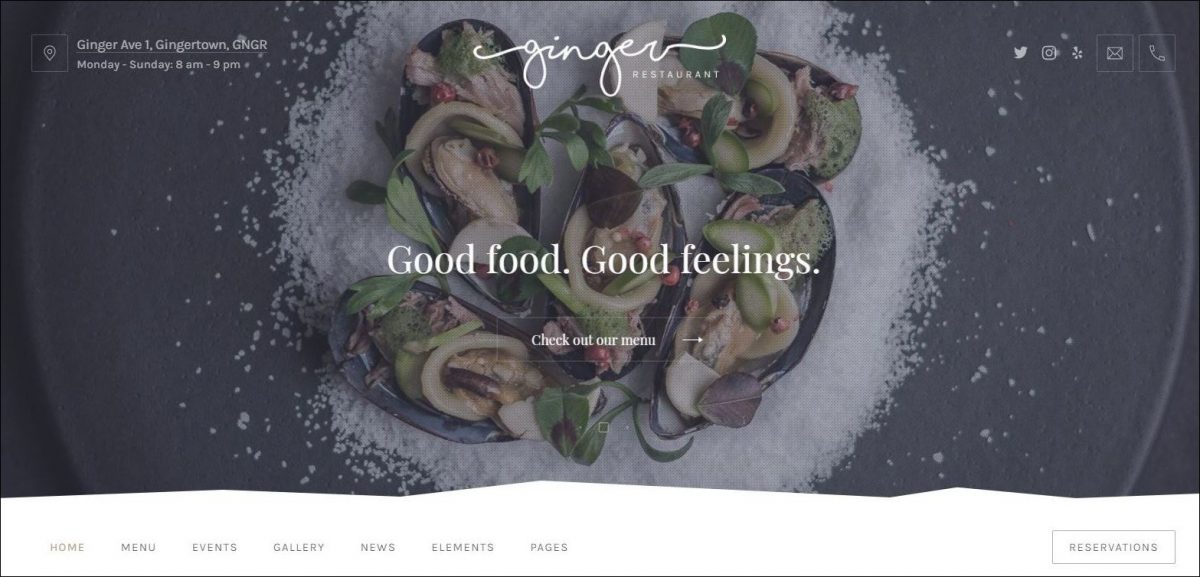Image Description for Ginger Restaurant Advertisement:

The advertisement for Ginger Restaurant features an elegant and curly script in the center that reads "ginger" in lowercase letters, reminiscent of the style of E.E. Cummings. The design is delicate and artistic, enhancing the visual appeal. The centerpiece of the ad displays an inviting image of gourmet food, possibly featuring a dish served on the half shell with avocado, enticing viewers with its fresh ingredients.

Below this visual, the tagline "Good food, good feelings" captures the essence of the restaurant's philosophy. A call-to-action button invites potential patrons to "check out our menus."

On the left side of the ad, you find important location details, which read "Ginger Ave, Ginger Town" alongside a stylized abbreviation "G-N-G-R." The restaurant's operational hours are also clearly listed: "Monday to Sunday, 8 a.m. to 9 p.m.," indicating that they are open every day of the week.

A small icon near the location information appears to resemble a hot air balloon, possibly offering directions to the restaurant. 

In the upper right corner, a set of social sharing icons is featured. These include:
- Twitter (represented by its familiar bird icon)
- Instagram (a circular icon within a box)
- A snowflake-like symbol (unclear purpose)
- An envelope (for email)
- A landline telephone handset (likely for making a call)

At the bottom of the advertisement, a navigational menu offers links to "Home," "Menu," "Events," "Gallery," "News," "Elements," and "Pages." These options provide easy access to various sections of the restaurant’s website.

Finally, in the bottom right corner, there’s a box labeled "Reservations," encouraging visitors to secure a table in advance. This feature might be particularly useful for ensuring a spot during busy times or earning potential bonus offers for booking ahead.